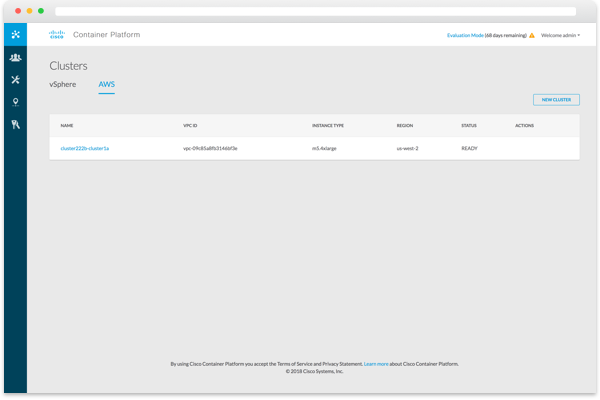The image displays a Cisco website, distinguished by a banner at the top, indicating it's a Cisco page. On the left side, there is a dark blue vertical menu featuring five selectable icons. The first icon, resembling an asterisk, is selected. Upon selection, a wide white rectangular bar appears, extending almost across the entire screen. This bar features the Cisco logo accompanied by the text "Cisco Container Platform." To the right of this bar, there are several dropdown menus and a small yellow triangle, though the text within them is too small to read. Beneath the "Cisco Container Platform" title, the word "Clusters" appears, offering two options: "vSphere" and "AWS." The user has selected "AWS," which has triggered an additional submenu to appear below it.